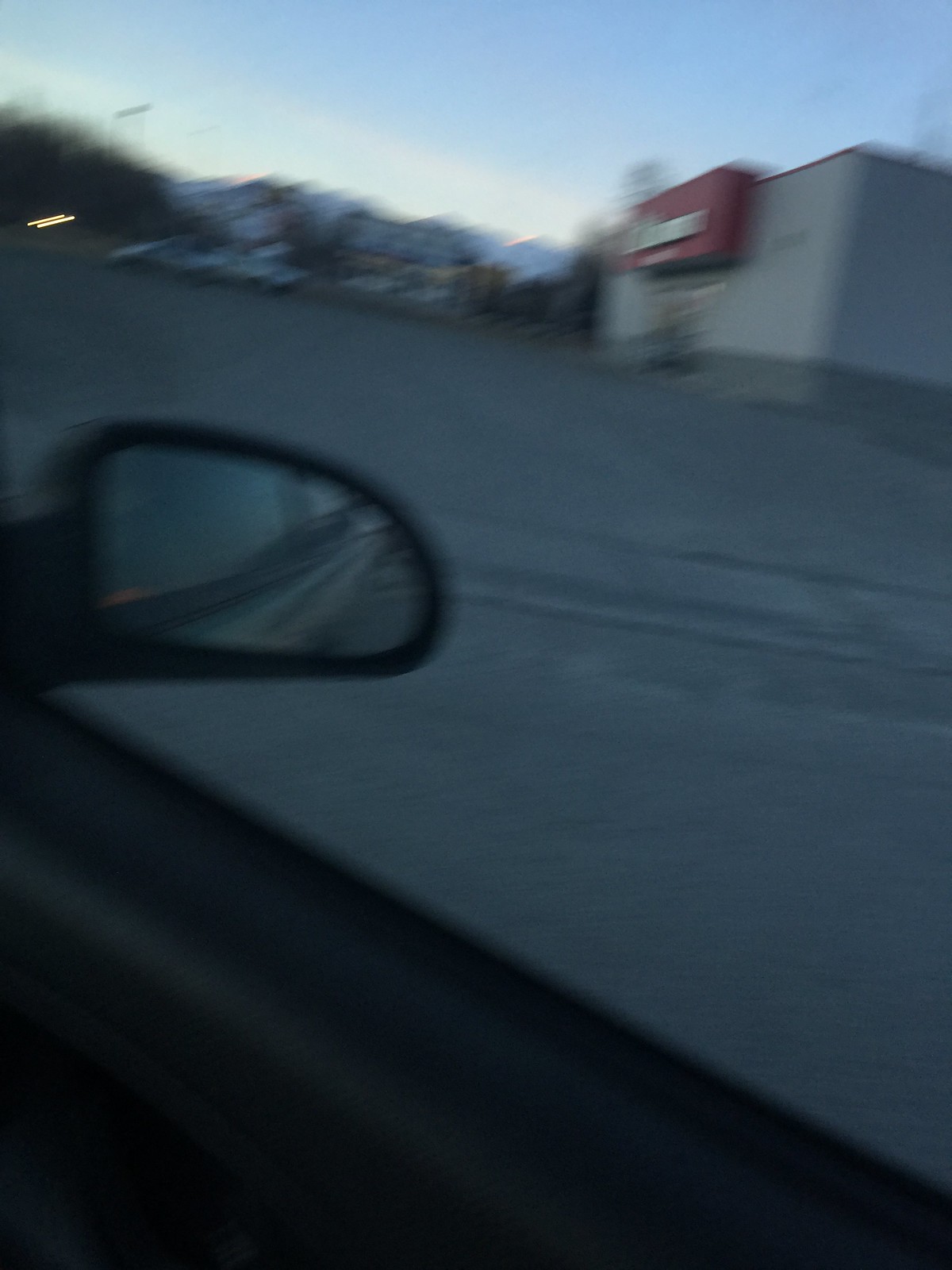The image, though notably blurry, is taken from the driver's side perspective inside a black car. The bottom of the frame reveals part of the car door. On the left side of the photo, the reflection of a car's back window and a partial view of its body is visible through the passenger side window. The scene outside showcases a fairly empty parking lot paved with gray cement or asphalt. In the background, to the left, there are two silver cars parked. To the right, a large building with white walls and a red accent above its entrance stands prominently. The building, likely a store, features illuminated letters and has lights on inside, suggesting it is afternoon and the daylight is still apparent. Additionally, there is a blurry billboard or building visible further back. The backdrop includes trees on the left and distant mountains, which are also blurry, under a clear blue sky.